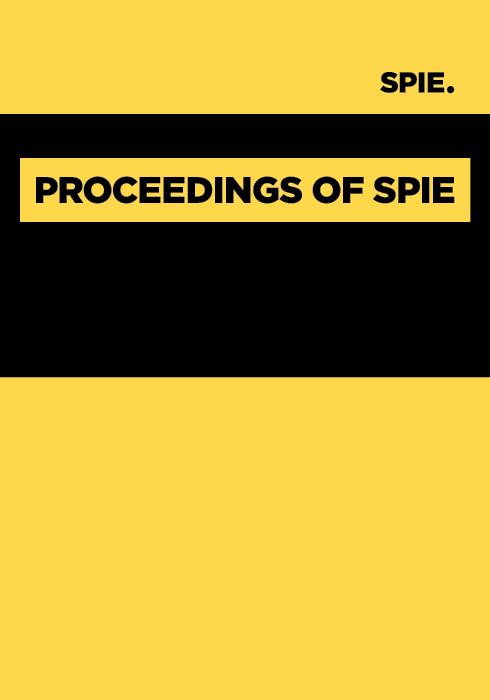The image is a book cover set against a yellow background, featuring a distinct horizontal black rectangle positioned around the middle. At the top right corner, in black text, it spells out "SPIE.", emphasizing the professional and academic nature of the publication. Within the black bar, there is a smaller, elongated yellow section running from left to right containing the title "Proceedings of SPIE" in larger black font. The design balances bold contrasts and clean lines, clearly segmenting the title and institution name against a simple, tricolor background.